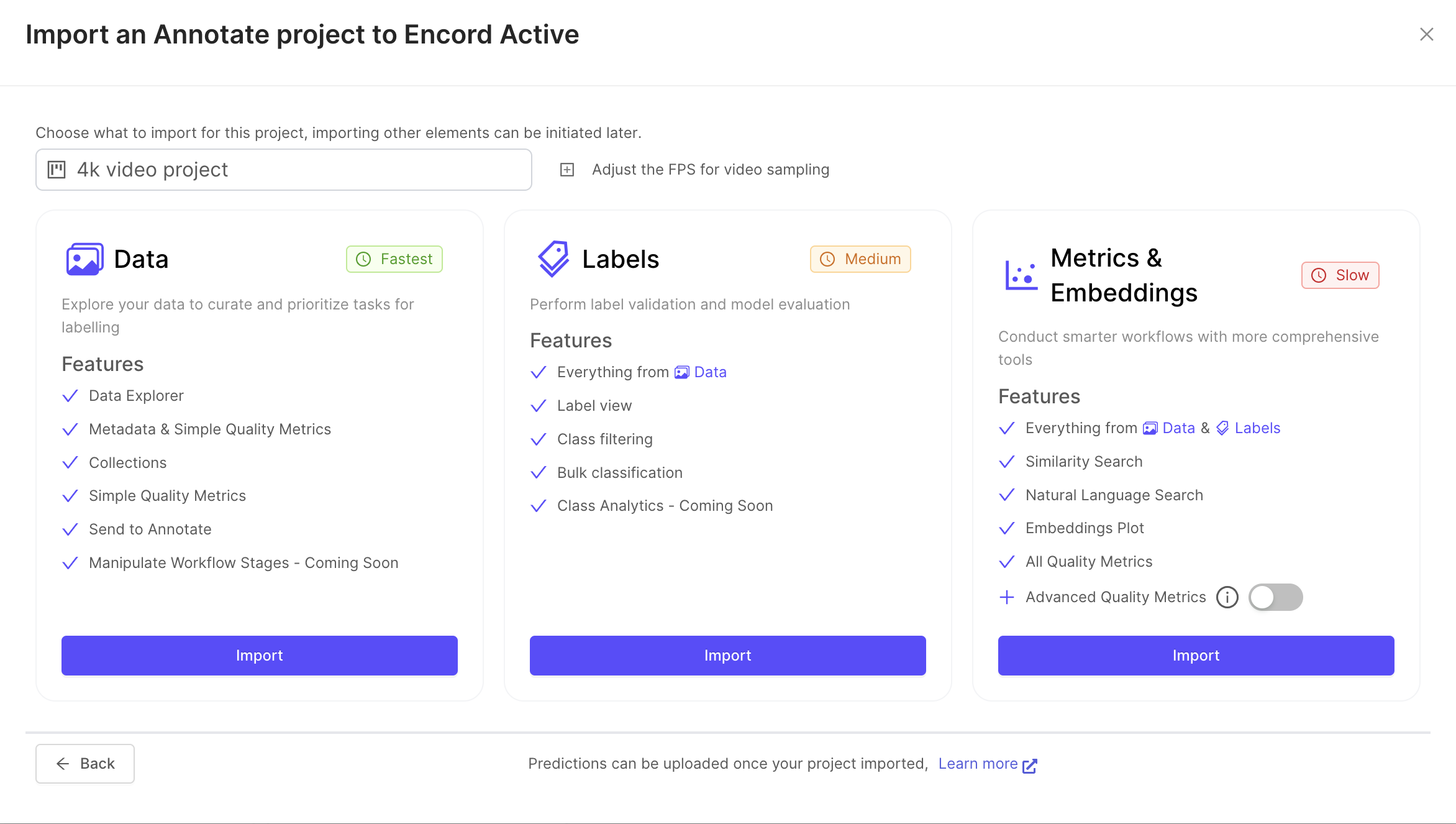The website interface is quite mundane and features a prominent notification for importing and annotating a project in an 'n-chord active' mode, displayed in black font. A faint line separates this section, followed by a small, light font instruction: "Choose what to import for this project. Importing other elements can be initiated later." Below this, a box labeled "4K Video Project" is accompanied by an option to adjust the FPS for video sampling.

The interface is divided into three main columns or boxes: Data, Labels, and Metrics & Embedding. Each section has listed features with corresponding check marks and a blue bar at the bottom with the word "Import" in white at the center.

At the very bottom of the interface, there is a line with a back button on the left, characterized by an arrow pointing to the left. Adjacent to this button, the sentence "Predictions can be uploaded once your project is imported" is displayed, followed by a "Learn More" link in blue font with an arrow icon. Another line further divides this section.

In the Data column, marked by a blue or green "Fastest" box, there is a description: "Explore your data to curate and prioritize tasks for labeling." The features listed with check marks include:
- Data Explorer
- Metadata and Simple Quality Metrics
- Collections and Simple Quality Metrics
- Send to Annotate
- Manipulate Workflow Stages (Coming Soon)

In the Labels column, labeled with an orange "Medium" box, the description reads: "Perform label validation and model evaluation." The listed features with check marks include:
- Everything from Data (Data is highlighted in blue)
- Label View
- Class Filtering
- Bulk Classification
- Class Analytics (Coming Soon)

In the Metrics & Embedding column, labeled with a red "Slow" box, the description states: "Conduct smarter workflows with more comprehensive tools." The listed features, all checked, include everything from Data and Labels (both highlighted in blue), along with:
- Similarity Search
- Natural Language Search
- Embeddings Plot
- All Quality Metrics
- Advanced Quality Metrics (marked with a plus sign and a special radio button next to it)

This detailed structure provides comprehensive options for managing various aspects of a project, from data import to advanced quality metrics evaluation.